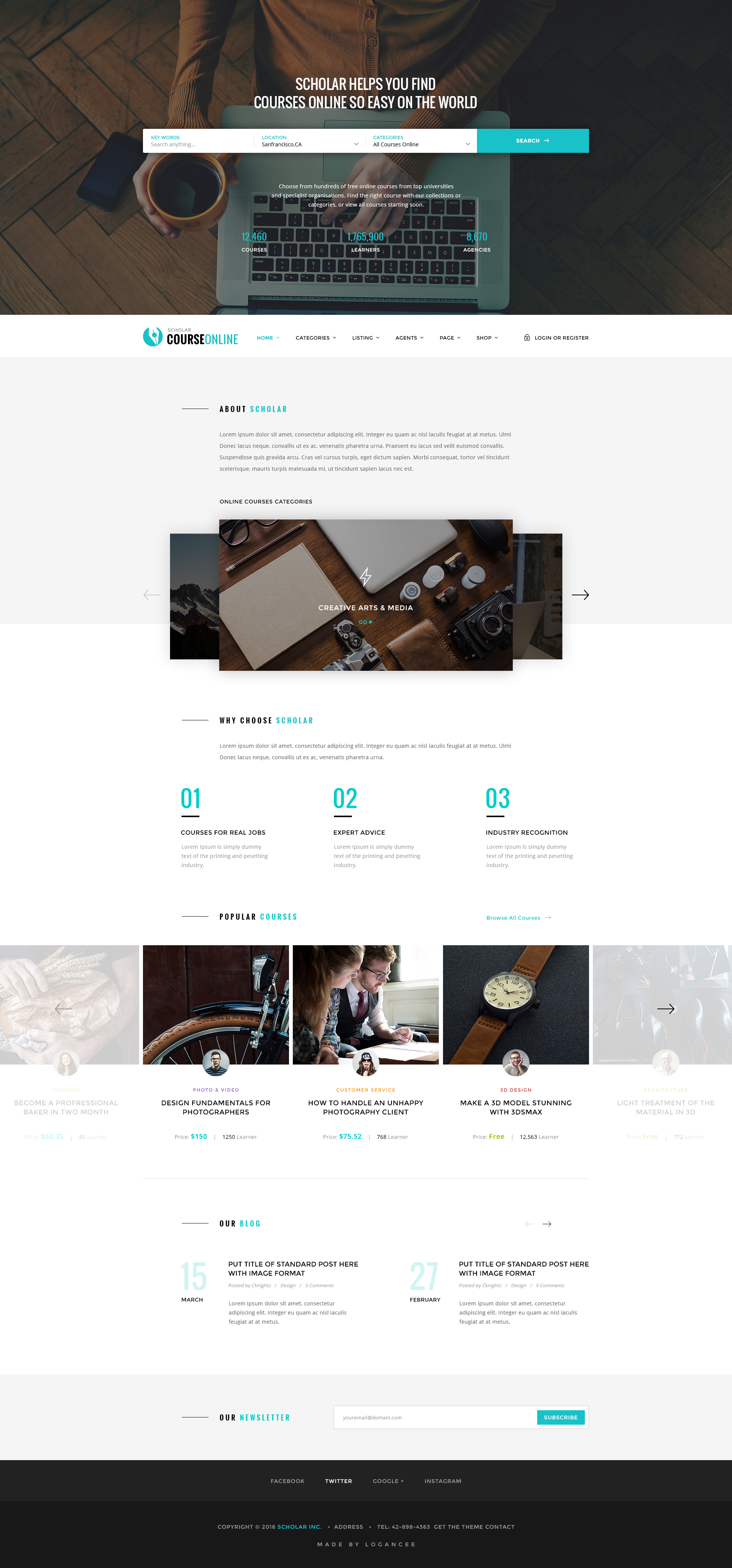The image depicts a webpage or application with extensive content, primarily showcasing an educational platform. At the top, there's a large banner featuring a bird's eye view photograph of someone using a MacBook laptop. The person, dressed in a brown cardigan, is typing with one hand on the keyboard while holding a cup of coffee in the other. Their phone lies on a parquet wooden floor. The photograph has a dark, moody tone.

In bold white text overlaying the banner, it reads: "Scholar helps you find courses online, so easy on the world." Below the banner is a teal-colored search bar where users can search by keywords, location, or course categories. Further down, text highlights the platform’s offerings: 12,460 courses, 1.7 million learners, and 7,600 agencies.

The remainder of the page transitions to a white background. The heading "Scholar Course Online" appears, followed by navigation options including Home, Categories, Listing, Agents, Page, Shop, Log In, or Register. Next comes an "About Scholar" section, with "Scholar" written in teal. This is followed by placeholder text (Lorem Ipsum).

Adjacent to this, an "Online Course Categories" section features icons for various creative fields: photography, film, a pencil, glasses, and paper, with the label "Creative Arts and Media" and a clickable "Go" button.

Another section, titled "Why choose Scholar?" lists three horizontally arranged points: 1. Courses for real jobs, 2. Expert advice, 3. Industry recognition. 

Following this is a "Popular Courses" segment, showcasing courses such as "Become a Professional Baker in 2 Months," "Design Fundamentals for Photographers," "How to Handle Unhappy Photography Clients," "Make a 3D Model Stunning with 3DS Max," and "Light Treatment of the Material in 3D," each accompanied by a relevant image.

Finally, there is a section about the blog with entries dated March 15th and February 27th.